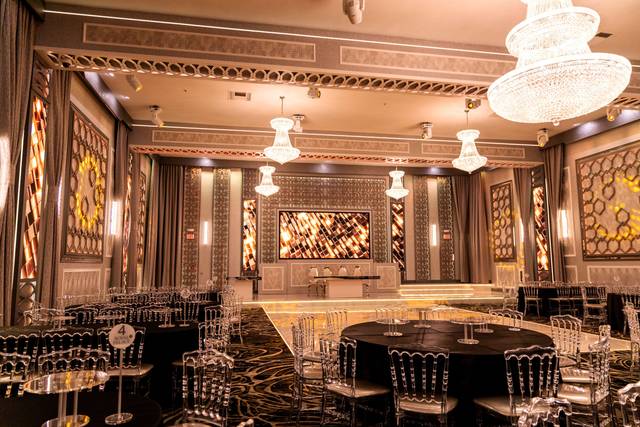The image depicts the interior of an upscale dining area, which could be a high-end restaurant or event hall, characterized by its elegant and sophisticated design. The room features at least five exquisite, tiered glass chandeliers casting a warm, light yellow glow, enhancing the cozy atmosphere. The ceiling is adorned with wooden beams and decorations against a rich brown backdrop. The walls are a mocha color, featuring intricate geometric patterns in shades of brown and gold, including diagonal and square shapes. In the foreground, there are round tables with dark tablecloths accompanied by chairs with silver backs and cushioned seats, as well as rectangular tables with black tablecloths. The tables are set with what appear to be trays and glass fixtures resembling cake holders, adding to the room’s opulent feel. A centrally located stage at the far end of the room, framed by more of the same geometric wall designs, suggests a space designed for performances or presentations. Along the sides, a carpeted area edges what seems to be a dance floor in front of the stage, hinting at the room’s versatility for events and gatherings.